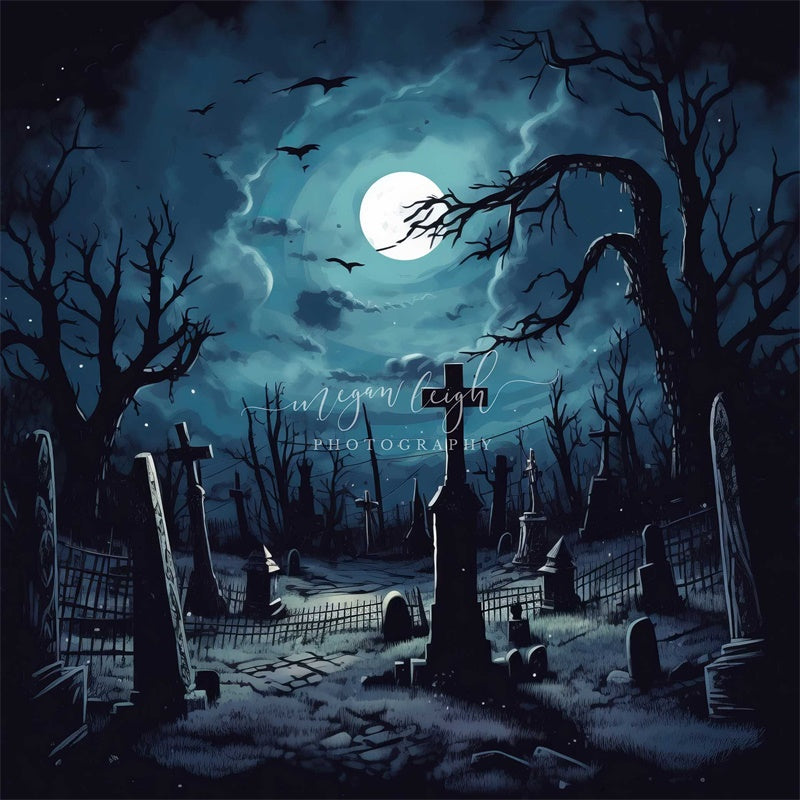A haunting illustration captures a cemetery bathed in eerie moonlight. The foreground features a prominently silhouetted headstone adorned with a cross, while various other tombstones, some topped with crosses and others with spires, stretch into the background. Looming to the sides are sinister, leafless trees, their twisted branches stark against a luminous, cloudy, blue night sky. A dilapidated black fence can be discerned among the shadows. The full moon, glowing brightly in the upper middle of the scene, casts a silvery light on the landscape, highlighting the silhouetted gravestones and scraggly trees. Black birds ominously circle the moon, enhancing the spooky atmosphere. A white script watermark reads "Megan Lee Photography," even though this is clearly an atmospheric painting rather than a photograph.